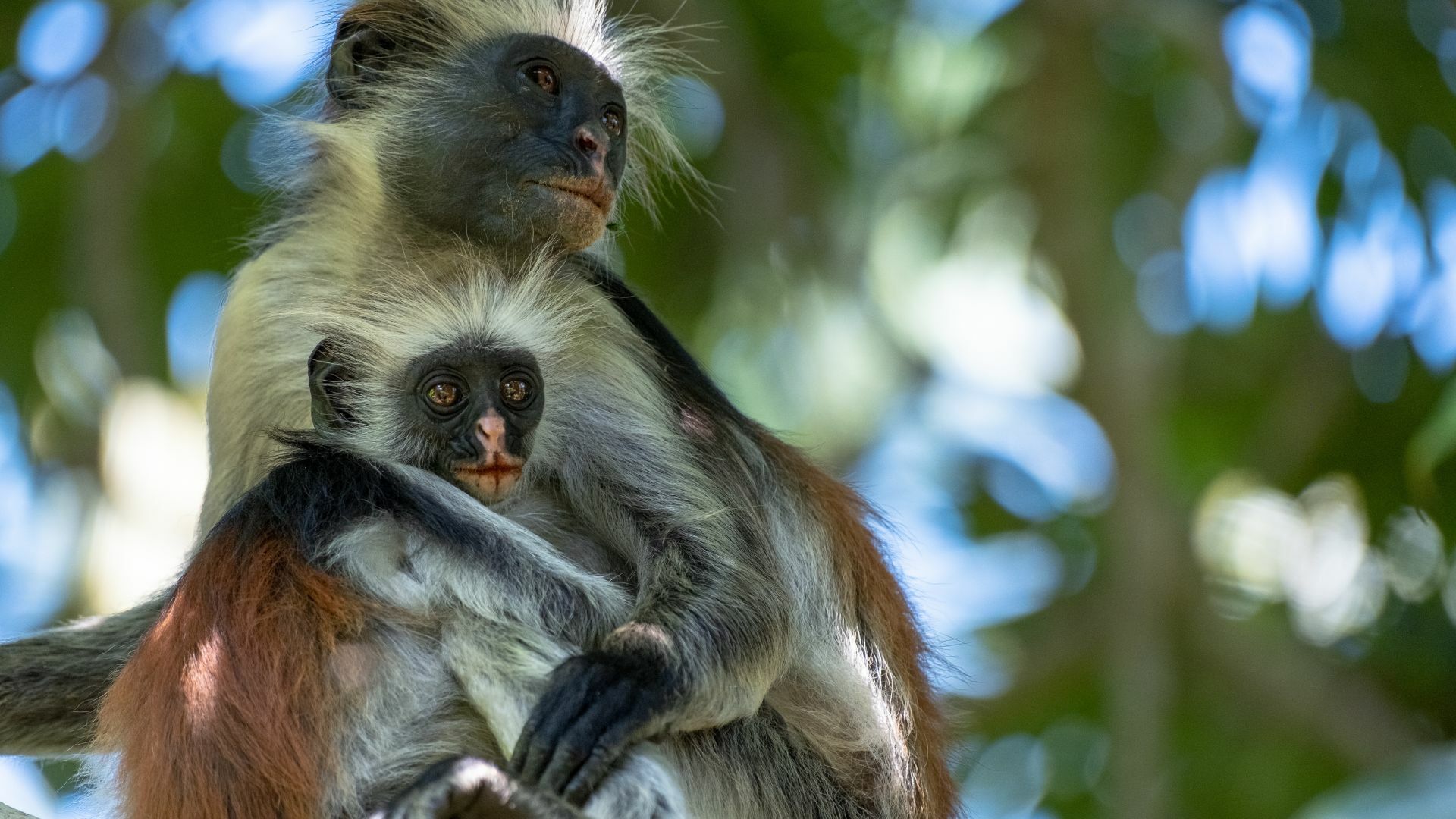The photograph showcases a heartwarming scene of a mother monkey cradling her young offspring while perched on a tree limb. Both monkeys feature distinct tiny black faces, large expressive brown eyes, and small pink noses. The mother's human-like black hand gently rests on the adolescent monkey's leg, who is snuggled close below her arm. They both have characteristic tufts of white fur atop their heads, while the fur on their bodies is a mix of whitish-gray and brown. Their backs display patches of light brown fur. The background is a blur of jungle trees with sunlight filtering through green leaves and branches, creating a serene and natural setting. The adorable pair exude a loving and protective aura as they gaze off into the distance, highlighting their unique bond and the beauty of their natural habitat.